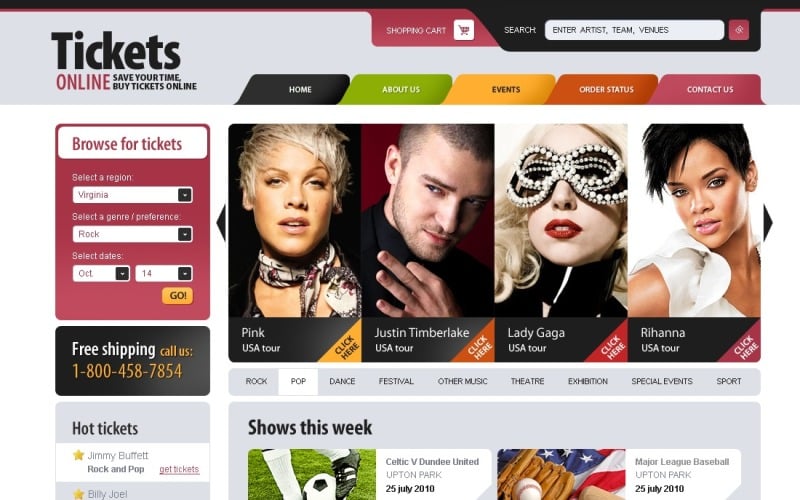The image features the homepage of an online ticketing website designed to save users time by enabling them to purchase tickets directly online. The top navigation bar includes buttons labeled "Home," "About Us," "Events," and "Contact Us." Below the buttons, smaller text prompts users to browse for tickets and search by region. A search bar shows the region "Virginia" selected, and a genre dropdown lists "Rock" as the chosen genre. The selected event date is October 14th, with a prominent "Go" button to proceed.

Key features also highlighted include free shipping and a customer support number. Beneath these details, a "Hot Tickets" section showcases popular artists such as Jimmy Buffet, Pink, Justin Timberlake, Lady Gaga, Rihanna, and Usher, encouraging users to "Get Tickets" for these shows. Various categories such as Rock, Pop, Dance, Festival, Other Music, Theatre, Exhibition, Special Events, and Sport are displayed, with special mention of an upcoming event, "Celtic vs Dundee United," scheduled for the current week.